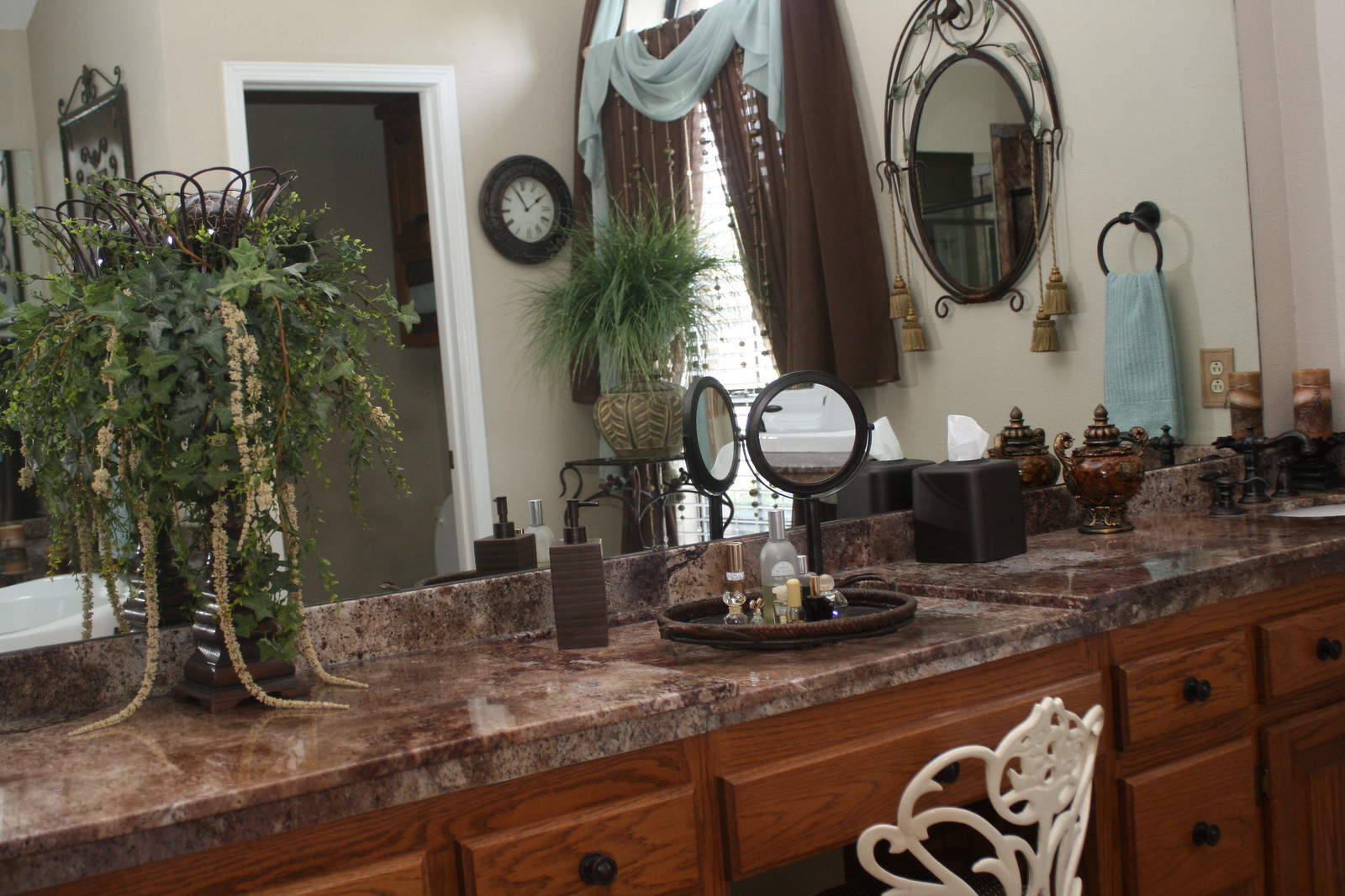The indoor bathroom image captures a neatly designed vanity area. On the left side, a lush hanging plant adorned with delicate white flowers or vines adds a touch of nature. A large mirror mounted on the back wall reflects the room, complemented by a granite countertop below it. The countertop is supported by a series of drawers made from walnut-colored wood, each adorned with black knobs, adding to the sophisticated look.

A pristine white chair is positioned in front of the vanity, inviting comfort. On the countertop, a vanity tray showcases an array of beauty essentials, including a mirror, various perfumes, and body splashes, epitomizing elegance and functionality. 

To the right, a stylish brown tissue box with a matching cover sits adjacent to a small vase. Another mirror is strategically placed on the right wall, enhancing the sense of space, while a window in the far right corner is dressed with a brown curtain elegantly topped by a white sash, allowing natural light to filter through.

The room is painted a clean white, adding to the airy and fresh atmosphere, while the doorframe seen in the mirror matches in color. To complete the scene, a decorative candle sits in the far right corner on a wrought iron base, featuring a blend of brown, white, and tan swirls, providing a cozy, ambient touch to the bathroom's décor.